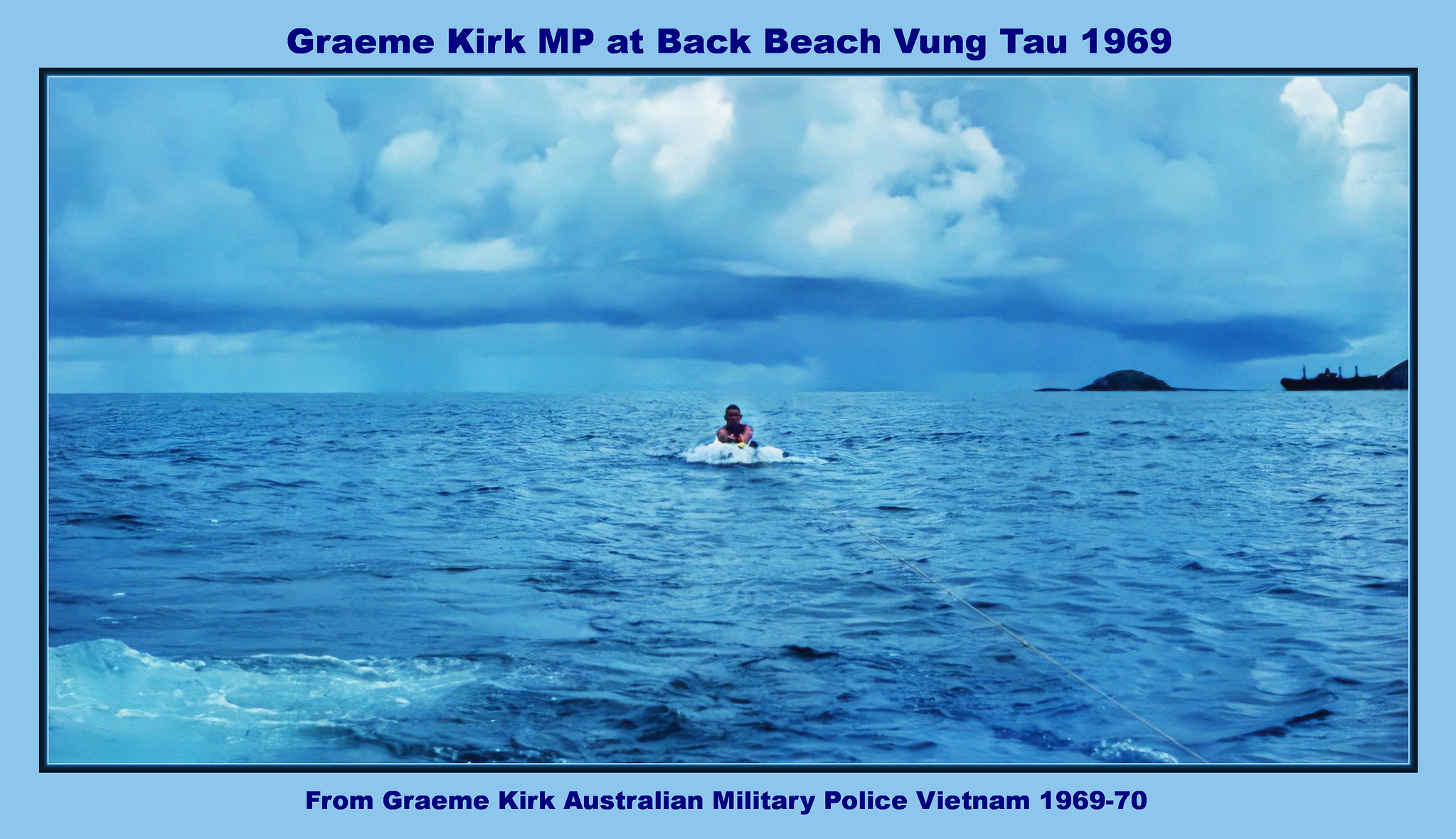This photograph, taken in 1969 at Back Beach, Vung Tau, Vietnam, captures Graham Kirk, a member of the Australian Military Police, skiing on the ocean. The sky is heavily clouded with white clouds, hinting at possible rain in the distance where some formations seem to emerge from the clouds. A mountain or hill and a black ship can be seen farther out on the horizon. Graham is engaged in water sports, holding onto a tow rope while being pulled by an unseen boat. The blue ocean is dotted with white waves, and the overall scene includes both the rugged natural landscape and the dynamic activity at the forefront. The image is labeled with "Graham Kirk MP" and notes the period of service as Vietnam, 1969-1970.